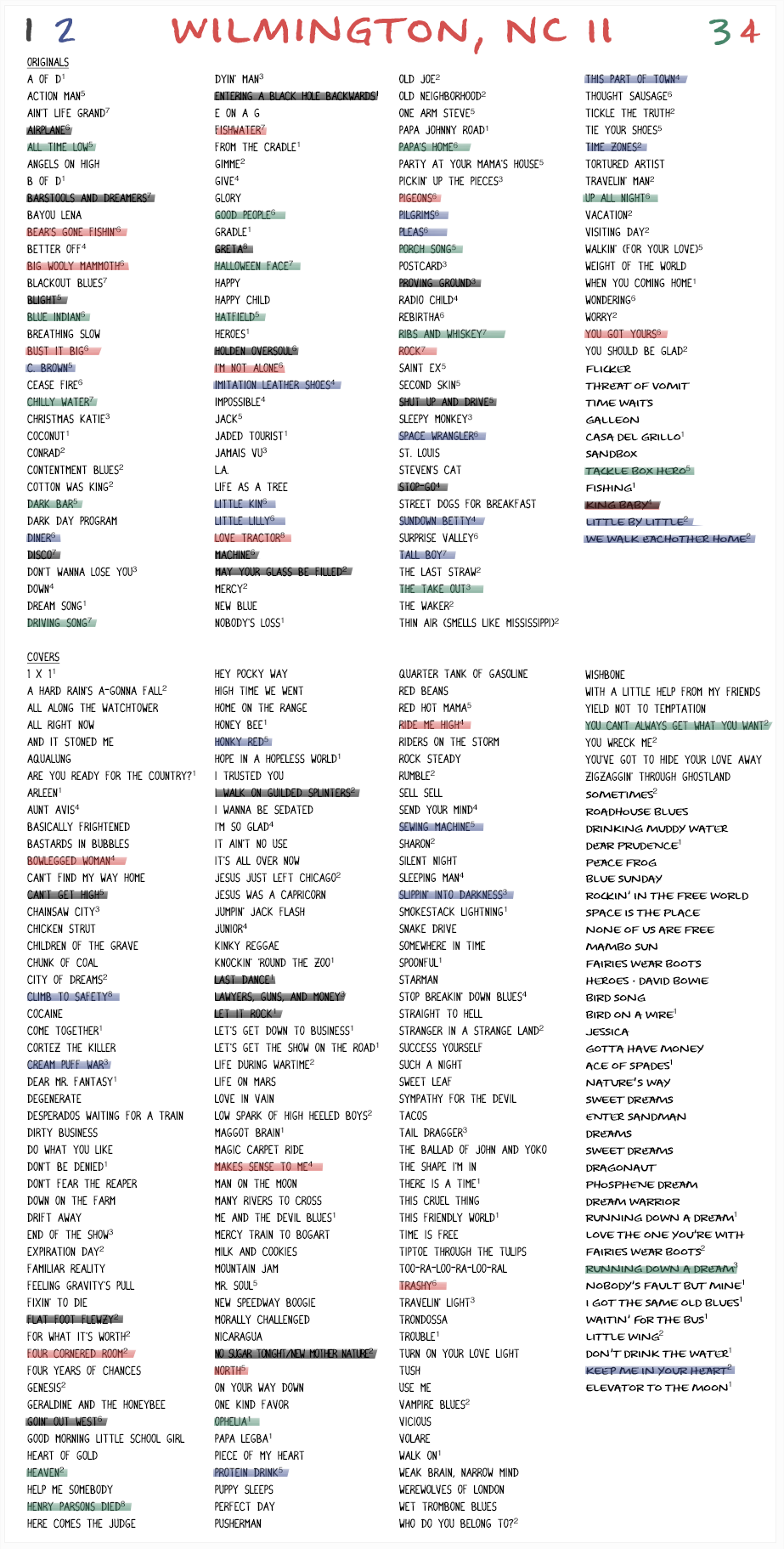The image features a stark white background with meticulously detailed elements scattered across its surface. In the upper left corner, the numbers "1" and "2" are prominently displayed, showcasing a handwritten aesthetic that could easily be mistaken for an artistic font. On the extreme right side of the image, the sequence "3-4" stands out with the number "3" rendered in blue and the number "4" in red.

Dominating the center of the image, the city name "WILMINGTON, NC" is presented in bold, all-caps, red font, clearly indicating Wilmington in North Carolina. Below this central text, the number "11" is discretely placed, adding another layer of detail to the composition.

Beneath this central section, the image is divided into four narrow columns filled with exceedingly small text, rendering it practically unreadable. Each column contains numerous rows of printed words, which appear to be a mix of potentially significant data such as temperature degrees and airport abbreviations. The precise nature of the text remains ambiguous due to its minuscule size, but the arrangement suggests a structured and detailed compilation of information.